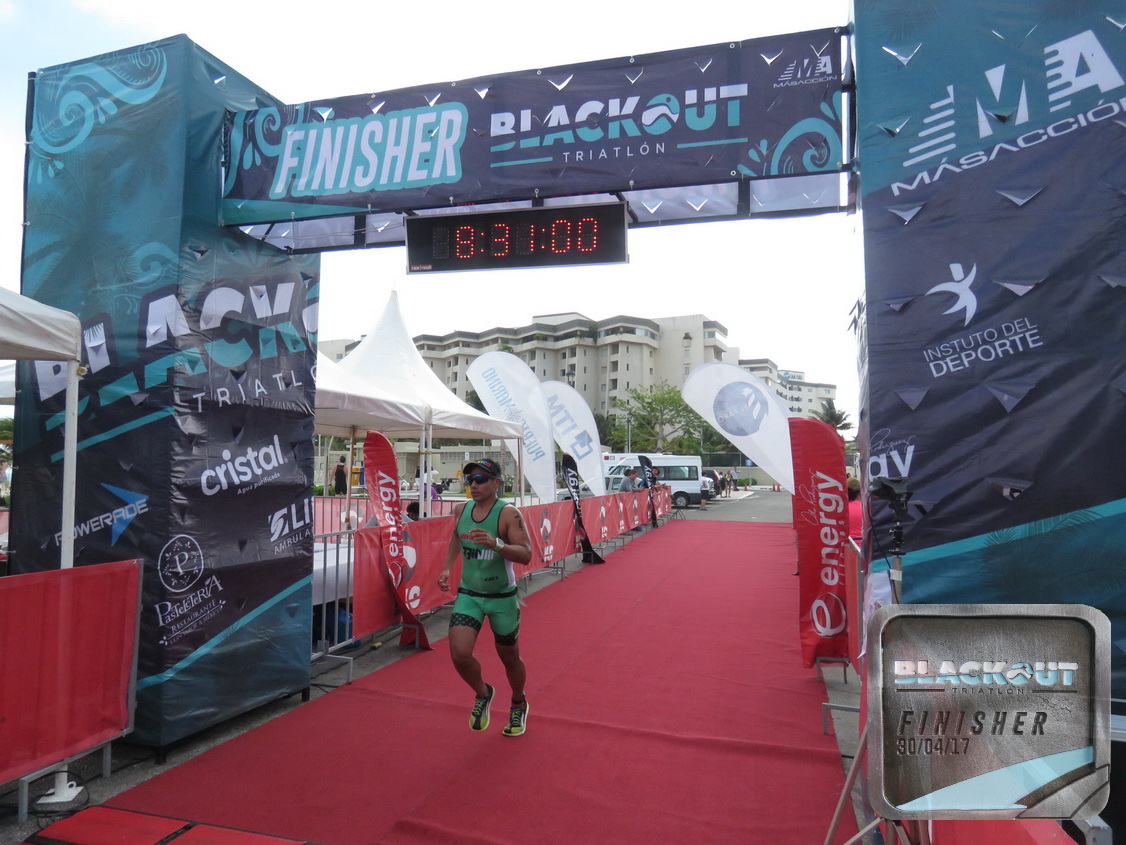An athlete crosses the finish line of the Blackout Triathlon, set against the backdrop of a towering structure that arches over the race's conclusion. The tower prominently displays the word "Finisher" and bears the logo of Instituto del Deporte, suggesting a Spanish-speaking locale. Sponsorship banners from Powerade and Cristal are visible, indicating their support for the event. The runner, clad in a green and black tank top and matching shorts, sports yellow and black tennis shoes. His recorded finish time is 8 hours and 31 minutes. Flanking his path are banners emblazoned with the word "Energy," adding to the vibrant and triumphant atmosphere. Notably, the red carpet under his feet enhances the moment of victory. The sparse crowd at the finish line leaves an open question as to whether he is among the front-runners or trailing behind the majority.